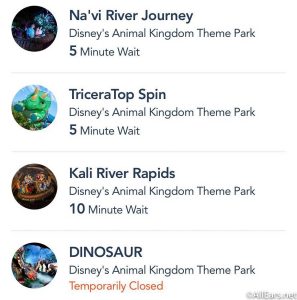This vertically-oriented rectangular image features four distinct sections, each separated by a thin gray horizontal line against a clean white background. On the left side of each section, there is a dark circle containing a small image, and on the right side, there is associated text with a title and brief description. 

- The top section's circle shows an image of two people, and the accompanying text reads: "**Navi River Journey**, Disney's Animal Kingdom theme park," with a note below stating a "5 minute wait."
- In the second section, the circle has an indistinct green figure, with the text next to it saying: "**Triceratop Spin**, Disney's Animal Kingdom theme park," also indicating a "5 minute wait."
- The third section presents a dark, brownish circle with an image that is difficult to discern. The relevant text states: "**Kali River Rapids**, Disney's Animal Kingdom theme park," noting a "10 minute wait."
- The fourth and final section features a circle with a somewhat vague blue and multicolor image. The text in this section reads: "**Dinosaur**, Disney's Animal Kingdom theme park," with the additional note "temporarily closed."

The structured layout and information provide a quick overview of these attractions and their status in Disney's Animal Kingdom theme park.